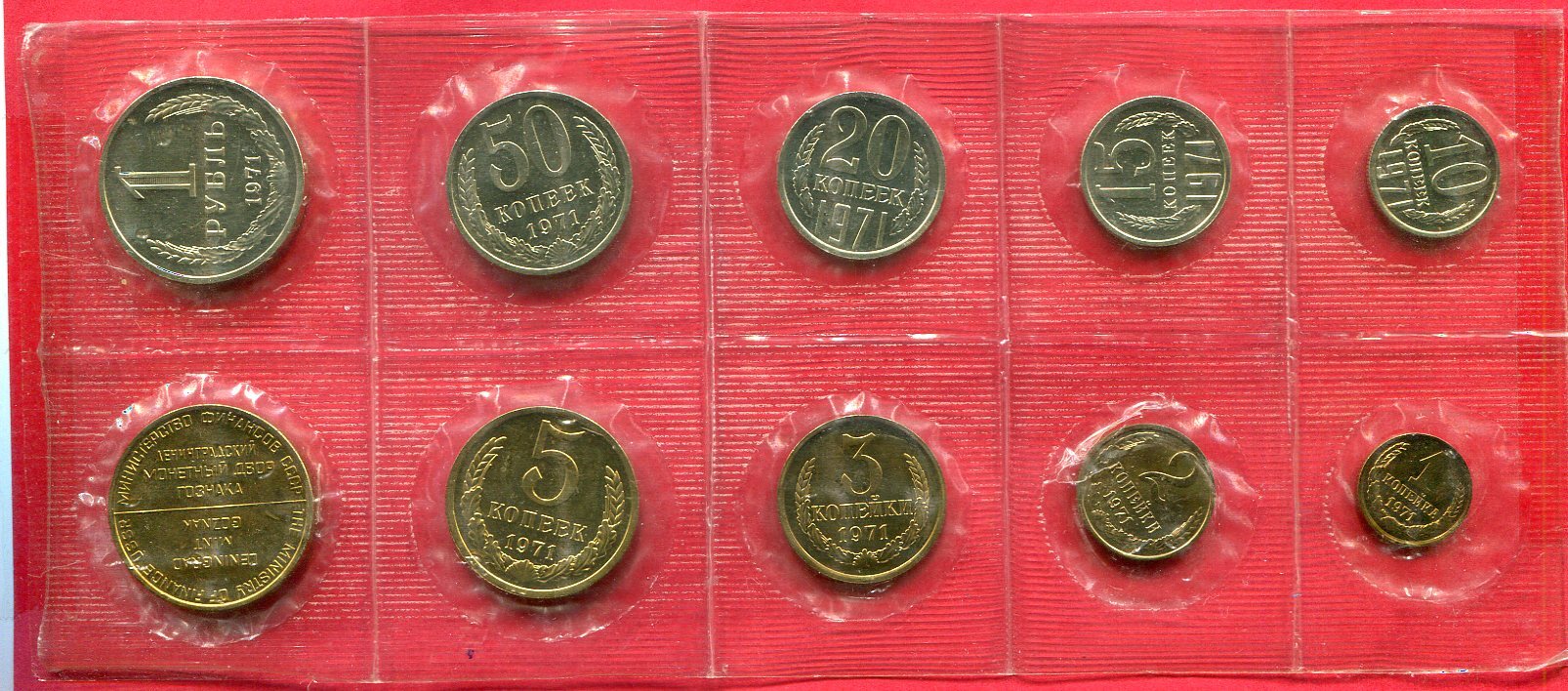This image presents a meticulously arranged collection of ten coins, each encased in a clear, horizontally textured plastic cover, framed against a thick, vibrant red background. The coins are secured to the backing, preventing them from being touched. The arrangement features two horizontal rows, with the top row displaying coins of a silver hue and the bottom row exhibiting coins of a brassy, bronze color. 

Starting from the top left, the first coin displays the denomination "1" followed by "1971." Adjacent to it is a slightly smaller coin marked "50," also from 1971, and the sequence continues with coins marked "20", "15", and "10," all from the same year. The second row showcases the reverse side of the first coin on the top left, followed by a brass-colored coin with the number "5" and the year 1971. Next, there are coins marked "3," "2," and the smallest coin with a "1," all also from 1971. The coins feature Russian lettering, indicating their origin, and the arrangement clearly demonstrates a decreasing size from left to right in each row.